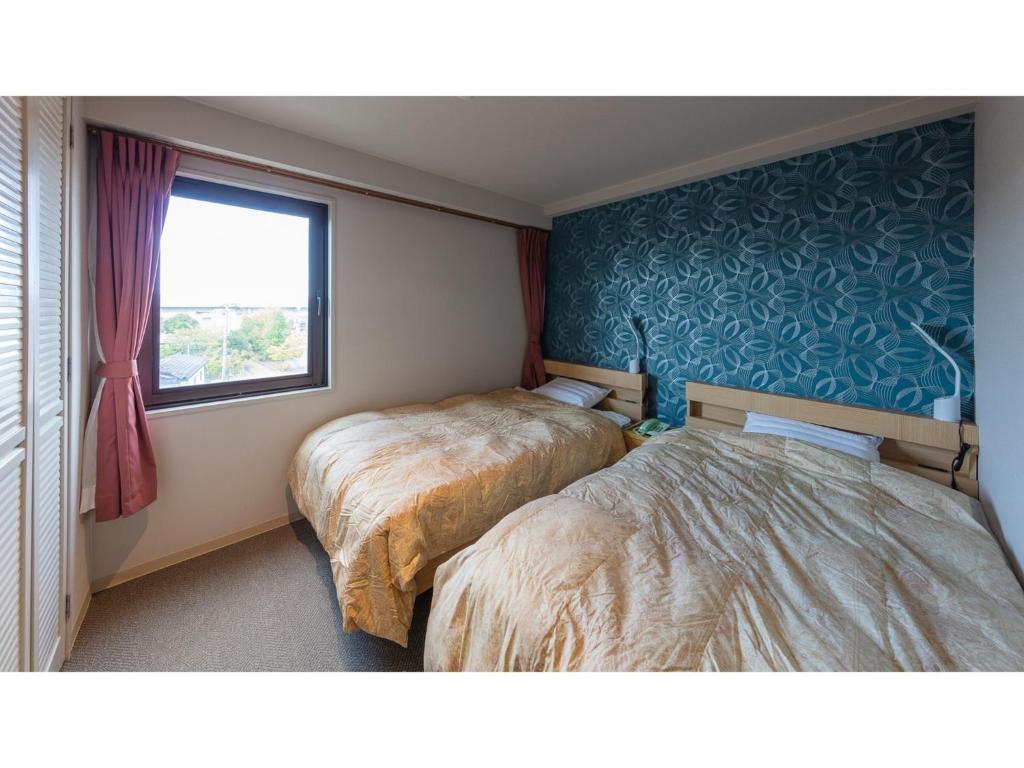This fisheye-view image, likely destined for an Airbnb or Travelocity listing, captures a cozy yet compact hotel room with twin double beds aligned side-by-side against a striking blue accent wall adorned with white geometric and floral patterns. Each bed, featuring wooden headboards, is dressed in cream or golden comforters with white pillows peeking out at the top. Small white lamps perched on the headboards create a symmetrical and inviting balance. Between the beds, a petite end table provides additional functionality. The room's left side showcases white sliding closet doors, while a nearby square window framed in black lets in an abundance of natural light, reflecting off the cream-colored walls. The window, adorned with pink curtains tied back into the room's corners, offers glimpses of an outdoor parking lot and another building bathed in sunlight. The floor is covered with a beige rug, adding warmth to this intimate space.